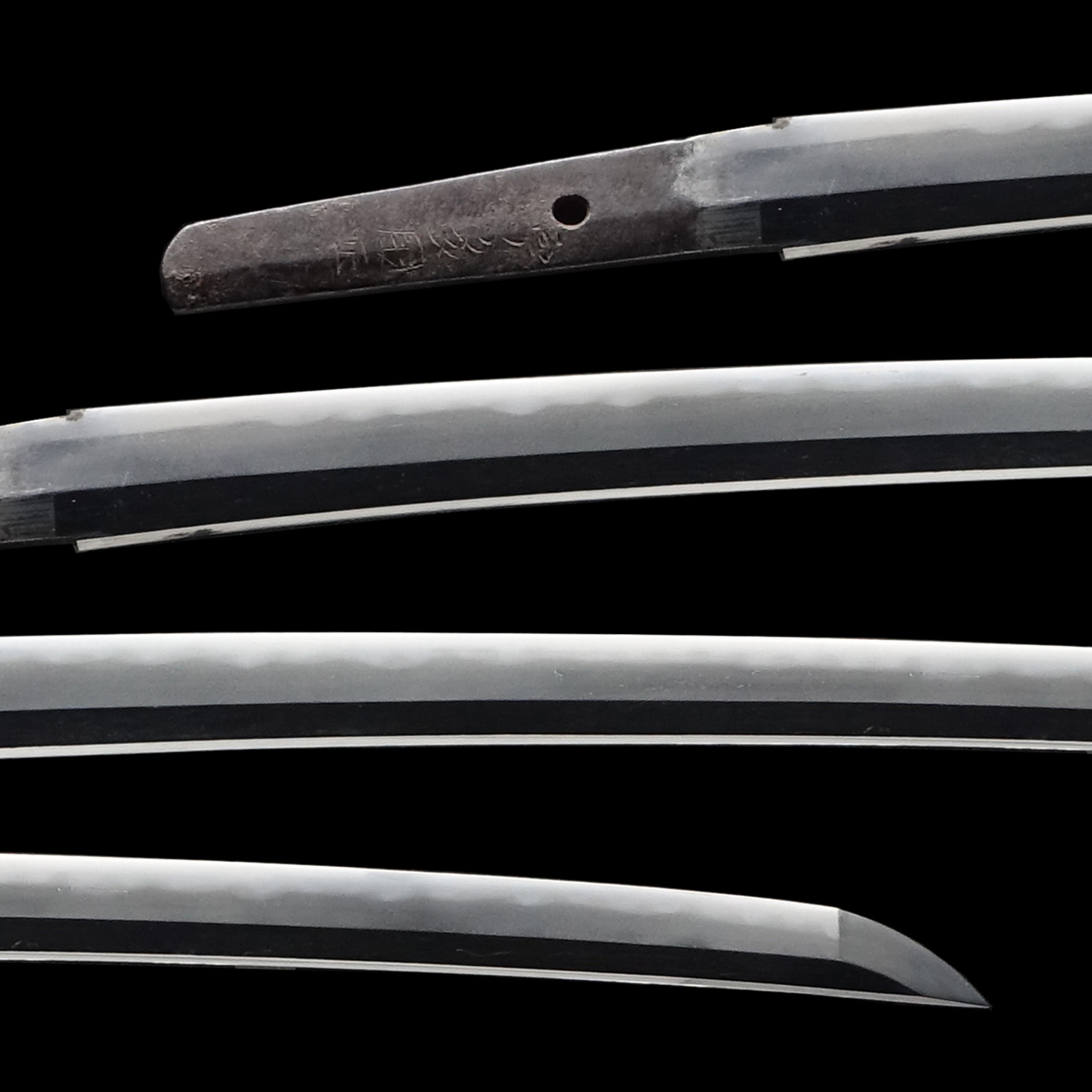The image displays four ancient Japanese swords, presented in sharp relief against a striking black background, emphasizing their silver hues. The swords are arranged in a row, and each one highlights different sections of the blade. The topmost sword is notable for its distinctive feature—a circular hole near the handle area, along with some Japanese lettering, although the exact details are unclear. This sword segment also indicates where a handle would be attached, though none of the swords have handles visible. The two central swords showcase only the blades, which are long, sharp, and well-preserved, exuding an aura of elegance. The bottommost blade displays its pointed tip, further emphasizing the fine craftsmanship. The entire arrangement, with its aged yet refined appearance, resembles an exquisite exhibit from a museum collection, possibly ancient samurai swords, drawing viewers' curiosity about their history and the significance of the hole in the top blade.